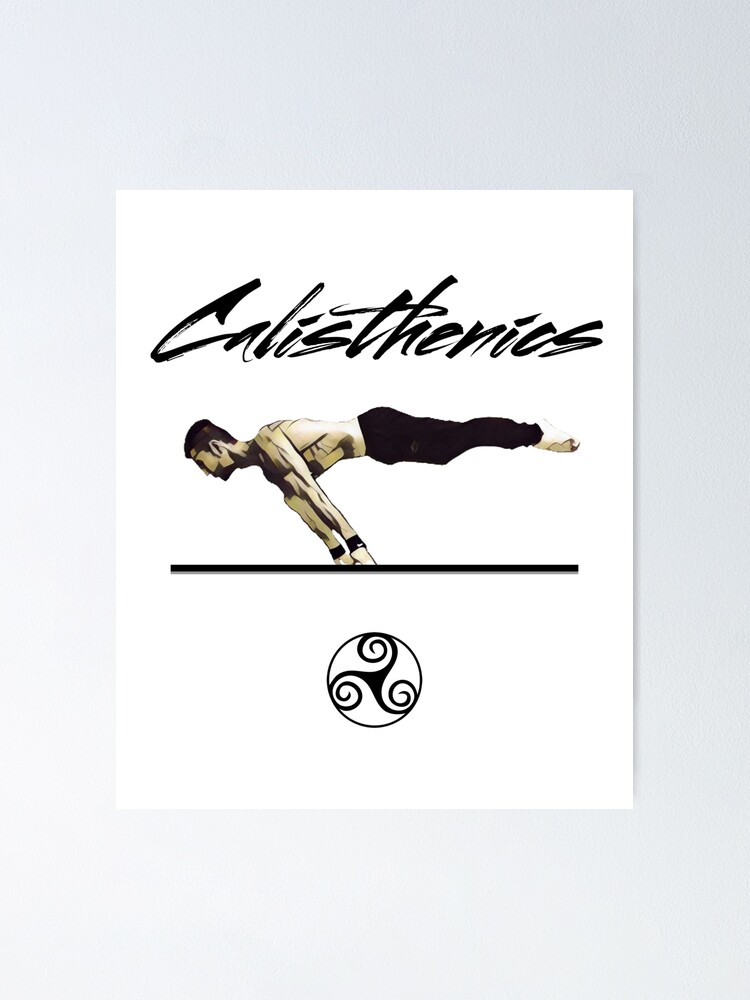The image depicts a digitally-drawn silhouette of a strong, muscular man performing a calisthenics exercise. Balancing on his fists, he maintains a plank-like position with his torso and extended legs elevated parallel to the ground. The man is clean-shaven, with black hair, no shirt, and black pants, hinting at his overall fit and well-defined physique. "Calisthenics" is prominently written at the top in a black, scribbled font reminiscent of marker writing. The background features shades of gray and white, giving the design a clean and modern look. At the bottom of the image is a circular logo with three swirl patterns, possibly representing the creator or brand behind the image.